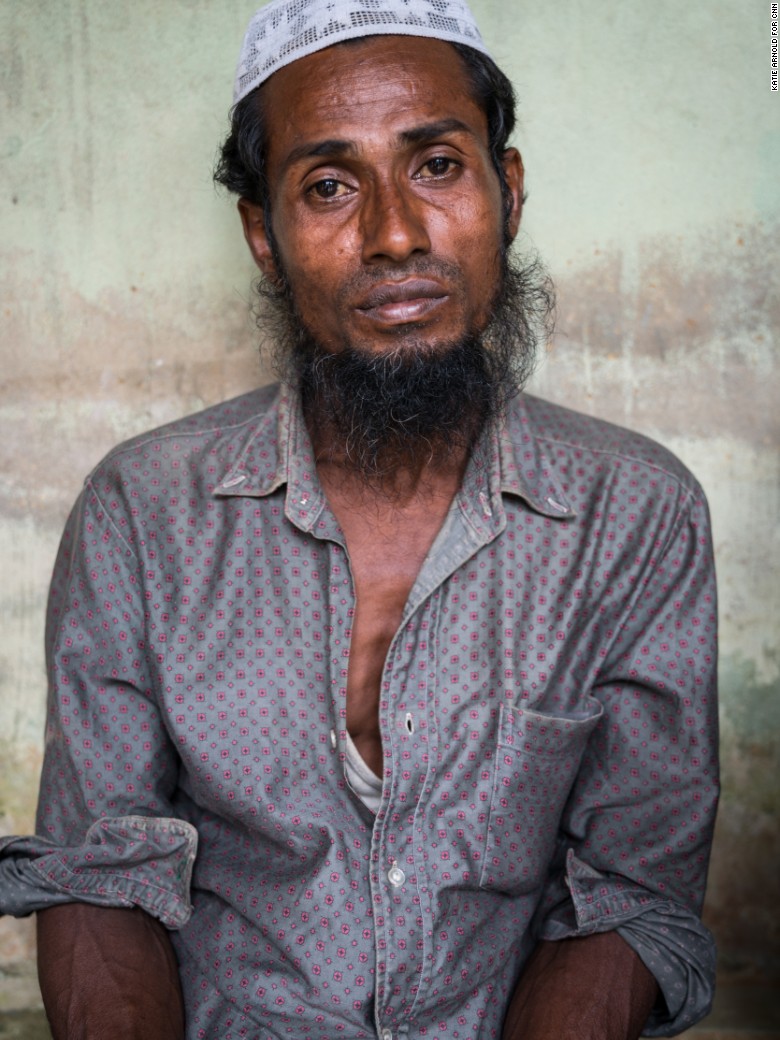A person, visibly exhausted, is seated against a somewhat grimy white stone wall with uneven patches of brownish-red staining its midsection. They are wearing a button-up gray shirt adorned with red dots, which is only buttoned halfway, partially exposing their chest and showcasing their veiny arms. Their short black hair is topped with a small white cap, and a wispy black beard frames their tired, sad face. Their sunburnt forehead adds to the appearance of weariness and despair. The overall ambiance of the scene emphasizes the person's melancholic state.